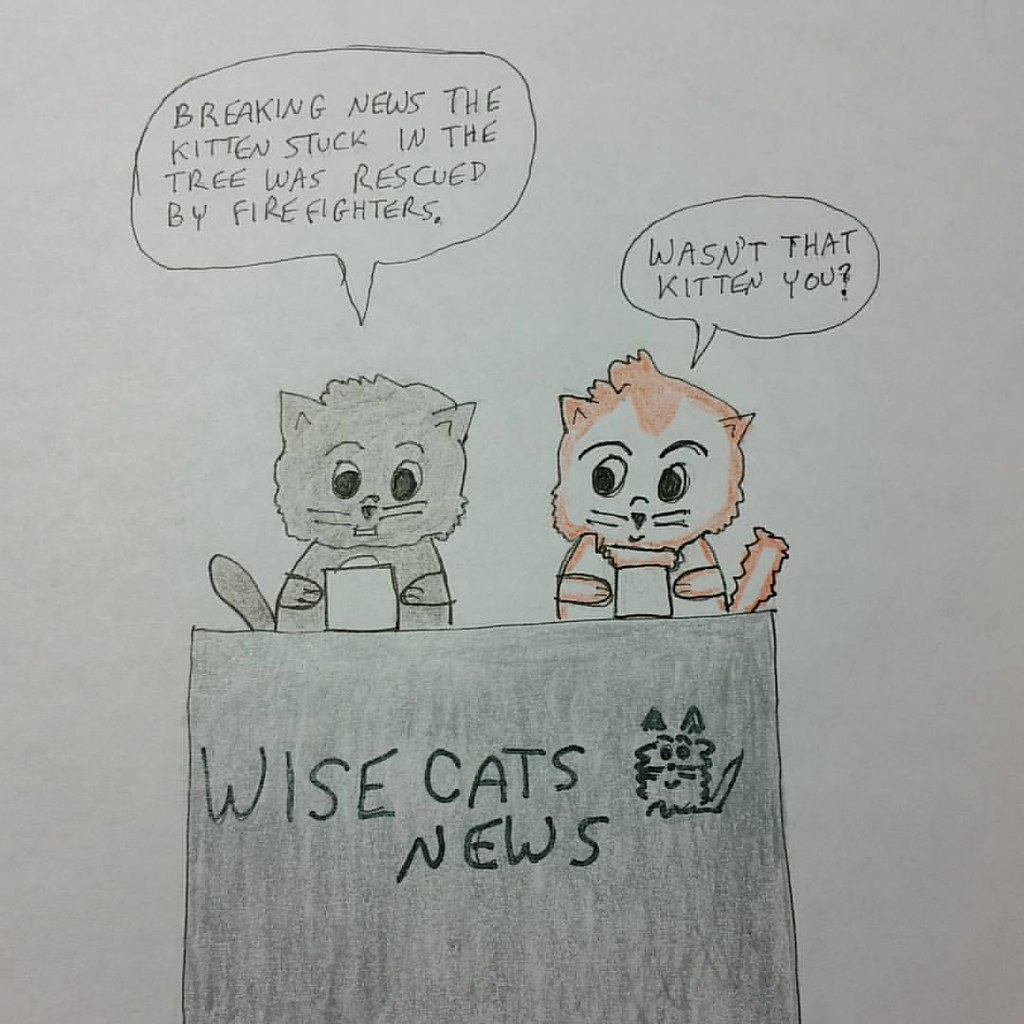This charming, hand-drawn cartoon features a whimsical news scene with two cat newscasters created on the back of an old piece of white paper using a blend of pencil, pen, and colored crayons. The background is a simplistic gray, drawing full attention to the animated characters and their comical exchange. The gray cat on the left is standing attentively, holding a piece of paper and looking down at it, while the orange cat on the right, accented with brown tones, looks towards the gray cat with a knowing expression, also holding some sheets of paper. Both cats are positioned behind a gray podium emblazoned with "Wise Cat News" and a small illustration of a cat. In the speech bubbles above their heads, the gray cat reports, "Breaking news, the kitten stuck in the tree was rescued by firefighters." The orange cat humorously retorts, "Wasn't that kitten you?" highlighting the playful joke of the gray cat reporting on its own past mishap. This delightful and quirky illustration captures the essence of innocent humor and creativity.